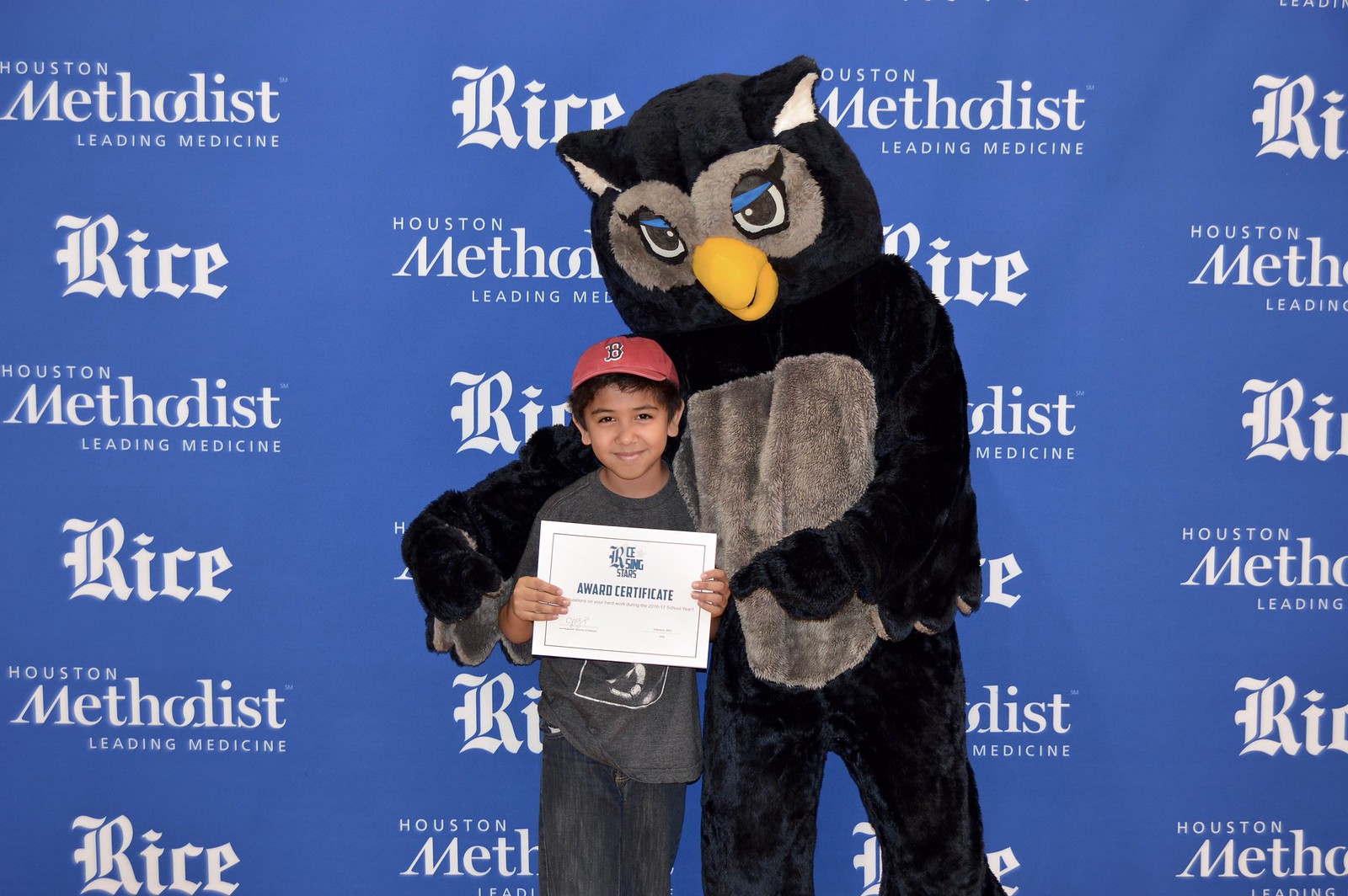In the large square image taken at an event, the background features a blue wall covered with the repeating words "Houston Methodist Leading Medicine" and "Rice" in white text, arranged in several columns. Centered against this backdrop is a mascot dressed in an owl costume, identifiable as the Rice University Owl. The owl costume is predominantly black with gray shading around the eyes and stomach area, blue upper eyelids, black eyes outlined in white, yellow beak, and black ears. The mascot has its right arm wrapped around a young boy, who is wearing a red Boston Red Sox baseball cap with a black letter "B." The boy is smiling and holding a white rectangular certificate with the words "Award Certificate" on it. He is dressed in a short-sleeve dark gray t-shirt and blue jeans. The owl mascot is pointing towards the certificate, while both pose for the camera.